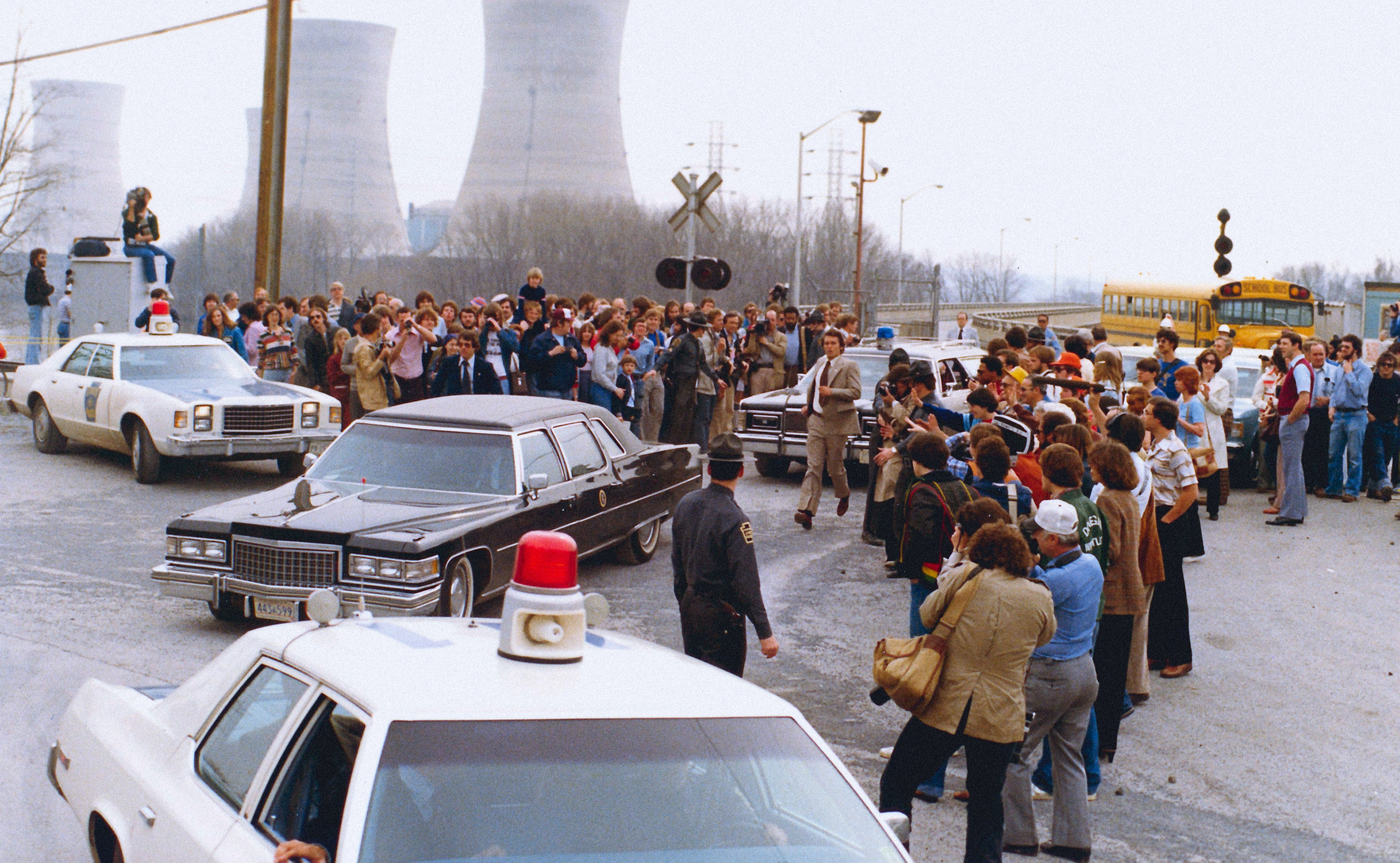In this detailed outdoor scene, a large crowd of people is gathered in the center of an asphalt road, directly in the middle of the image. The setting is reminiscent of the 1970s, with men and women dressed in era-appropriate clothing. Surrounding them are several cars, including clearly marked police vehicles with sirens, as well as unmarked government-type black cars that feature small, illegible emblems on their doors. In the foreground, a man in a suit is seen running toward a uniformed police officer, while media personnel with cameras capture the event. A school bus is parked in the distance, contributing to the bustling atmosphere. The backdrop features the iconic stacks of the Three Mile Island reactors, hinting at the historical context. Additionally, someone on the left side of the image is perched on a tall object, holding a camera. The vivid colors in the photo include tan, white, yellow, red, orange, black, gray, and blue, enhancing the lively midday, outdoor setting near a bridge.